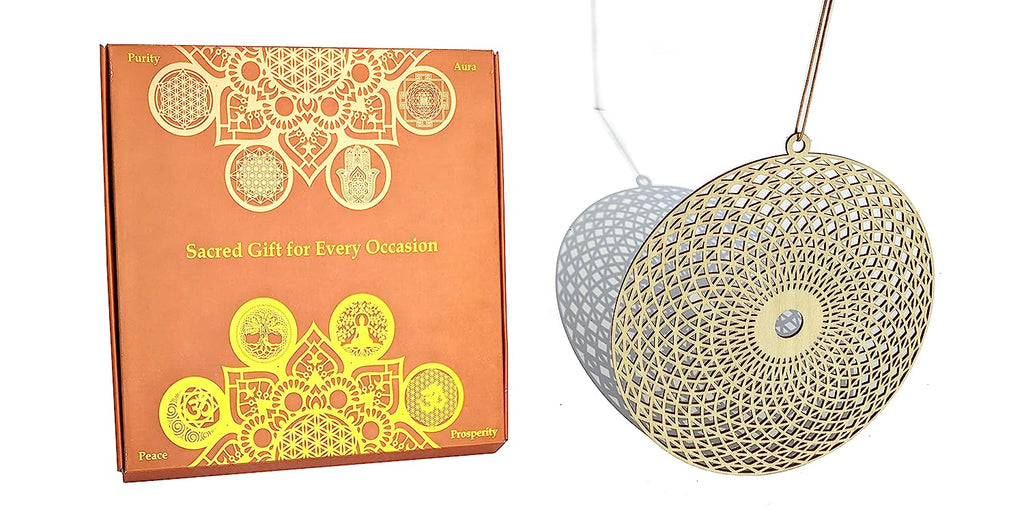The image features a square, rust-orange box decorated with an intricate mandala-like design in yellow and light gold. In the center, bold yellow text reads, "Sacred Gift for Every Occasion," with smaller text in each corner proclaiming "Purity," "Aura," "Peace," and "Prosperity" in matching yellow. The mandala design, with its webbed and ornate features, includes motifs such as leaf-like shapes, trees, and a person sitting down, with the number 30 appearing in several circles. To the right of the box, a detailed photo of a circular, gold metal pendant is displayed. The pendant features dense geometrical, curved lines creating diamond shapes, a solid ring around its hollow center, and an elaborate webbed, lace-like pattern. The pendant, designed to be worn on a string, casts a shadow that adds depth to the otherwise pure white background.